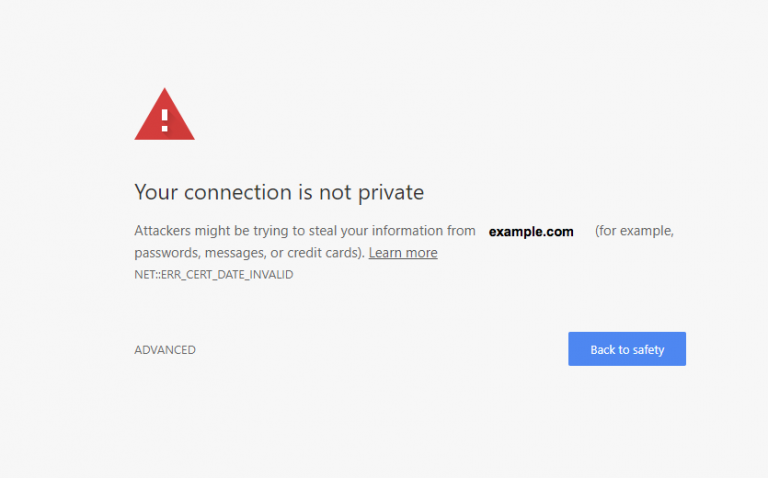A web browser security warning page is displayed prominently on the screen. At the top is a red triangle with a white exclamation point, indicating a cautionary alert. Below this icon, a bold message reads, "Your connection is not private." The warning further explains the potential risks: "Attackers may be trying to steal your information from example.com (for example, passwords, messages, or credit cards)." 

Additional text in a smaller font size states "NET::ERR_CERT_DATE_INVALID," suggesting that the site's security certificate is either out-of-date or invalid. This cryptic language informs the user about the technical issue behind the warning. 

The interface provides two buttons for proceeding: a prominent blue button labeled "Back to Safety," likely offering a safe retreat to the previous page, and a smaller "Advanced" button on the left. Clicking "Advanced" likely provides options to proceed to the site after being warned multiple times, stressing that the connection is potentially insecure.

The page's background is a light gray, and all text is rendered in black for clear visibility. The URL "example.com" is highlighted in bold, drawing attention to the specific site facing these security issues.